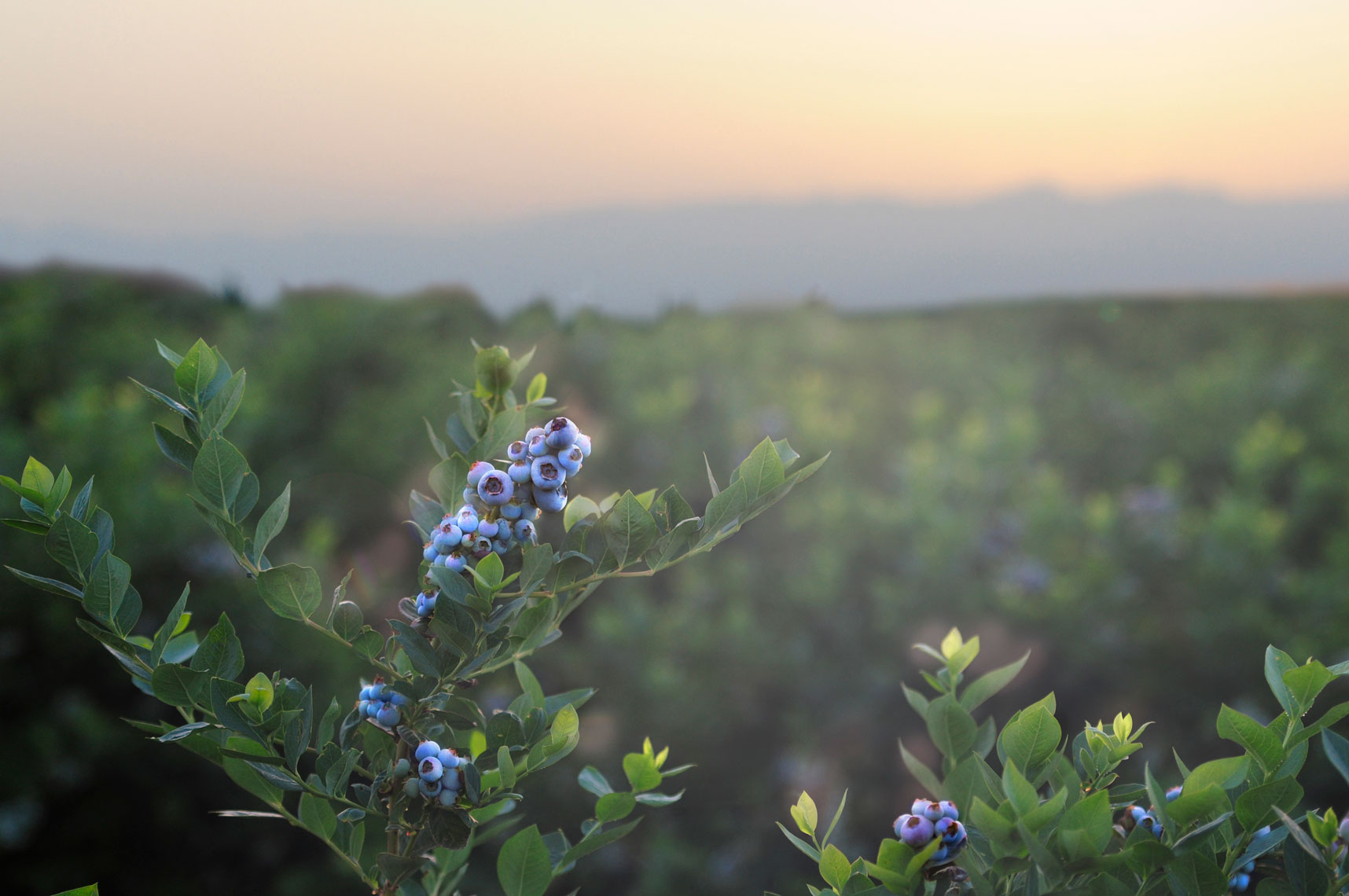The photograph is a rectangular image with the top and bottom sides twice as long as the left and right sides. It captures a vast berry field with a sharp focus on the foreground and a blurred background. In the foreground, multiple thin stems and branches of a berry bush rise from the bottom of the image. These stems, colored brown and green, are adorned with teardrop-shaped leaves that vary from dark to lighter green tones.

Prominently featured in the center and towards the top of the photograph are clusters of spherical blue berries, each with a small black blossom at the bottom, indicative of blueberries. Some clusters are large while others are smaller, containing fewer berries. Behind these foreground elements, the background reveals an expansive stretch of blueberry plants fading into the horizon. The foliage and additional berries become indistinct and blurry as they stretch back, suggesting the field extends far into the distance.

Above this lush expanse, the sky transitions from a light yellow at the top to a warm orange below, hinting at a setting sun. Across the horizon, a dark, blurry silhouette of hills or mountains runs horizontally, enhancing the depth and natural beauty of the scene. This picturesque nature photograph highlights the abundance and tranquility of the berry field under a serene sunset sky.